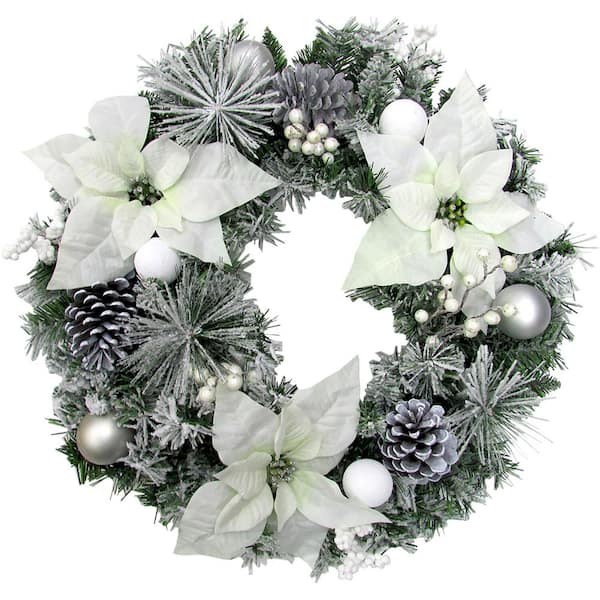This image depicts a standard-sized Christmas wreath, typically intended for a front door. The wreath consists of several plant parts, including spiky and flat leaves, with additional artificial green grasses. Prominently featured are pine cones, some of which have been painted silver but still reveal some brown underneath. The wreath is adorned with white poinsettia flowers: one at the upper left, one at the upper right, and one slightly to the left at the bottom. Each bloom has white petals and a green center.

In addition to the natural elements, the wreath includes various decorative accents, such as berries and silver Christmas orbs scattered throughout. Notably, there are white balls and silver bulbs enhancing its festive appearance, as well as spiny starburst-like ornaments. The green parts of the wreath suggest a frosted look, giving the impression of wintry trees dusted with snow. The center hole of the wreath is slightly irregular due to some of the greenery and poinsettias extending into it. With its mix of traditional and frosted elements, the wreath captures the essence of a wintry Christmas decoration.